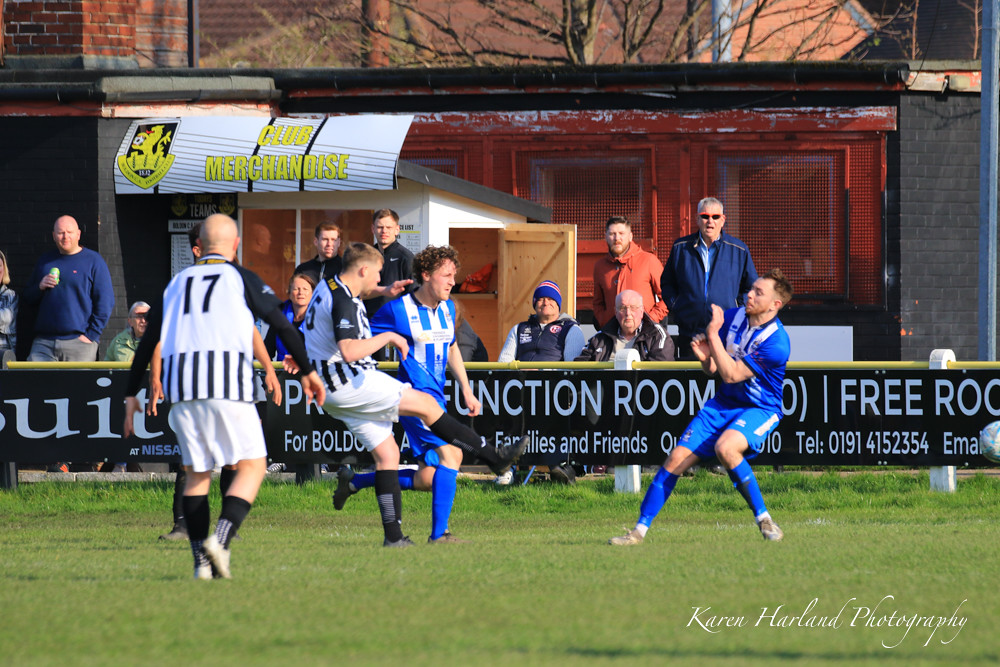In a sunny daytime image of an active soccer match, players from two opposing teams on a lush green field are intensely engaged. A player on the right, clad in a blue and white uniform, is crouched and appears to be clutching a barely visible blue ball in front of him. On the left, three players are seen, with one in a white jersey (number 17) with blue sleeves. The player in front of him, also in a white and blue jersey marked with the number five, has his right leg raised, poised to kick. The teams are distinguished by their uniforms: one in blue with white stripes, blue shorts, and socks; the other in white with black stripes and white shorts. 

In the background, a short barrier fence adorned with advertisements, including telephone numbers and company names, separates the field from a mixed crowd of seated and standing spectators. Above them, a sign reading "Club Merchandise" and an adjacent, blurry logo denote a small shack selling team goods. Further back, brickwork and a red building can be seen amongst the trees. Additionally, the lower right corner of the image is marked with the watermark "Karen Harland Photography."